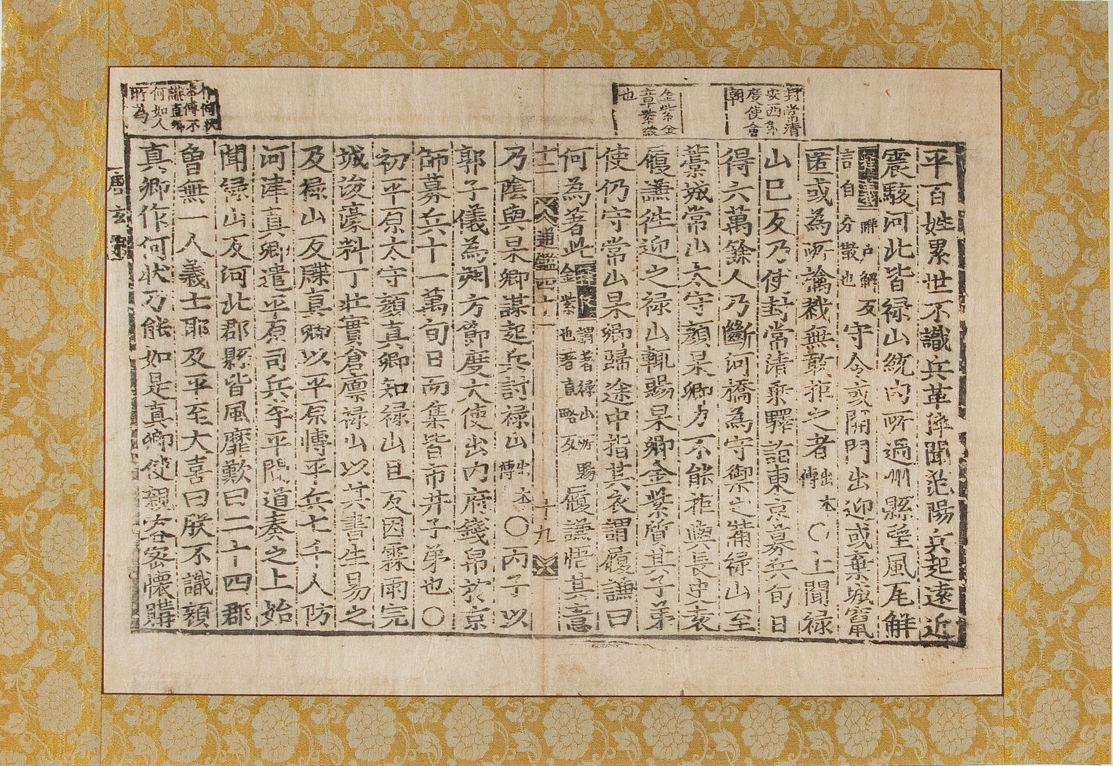The image depicts an aged piece of parchment or paper with a muted, pale appearance, covered entirely in black Japanese or Chinese characters, organized in numerous columns. It rests against a yellow background adorned with a repeating white floral design. The parchment itself, possibly having been folded at some point, has a slightly darker hue compared to the background. There are no titles or headings above the columns, just row after row of detailed lettering. At the top of the document, there are some stamped areas or boxes, suggesting it might be an official document or chart, possibly used in educational settings. The parchment appears to be centrally placed on the yellow floral mat, and the characters, grouped in columns numbering potentially between 12 to 20, provide an intricate and orderly display, though their exact message remains unreadable.